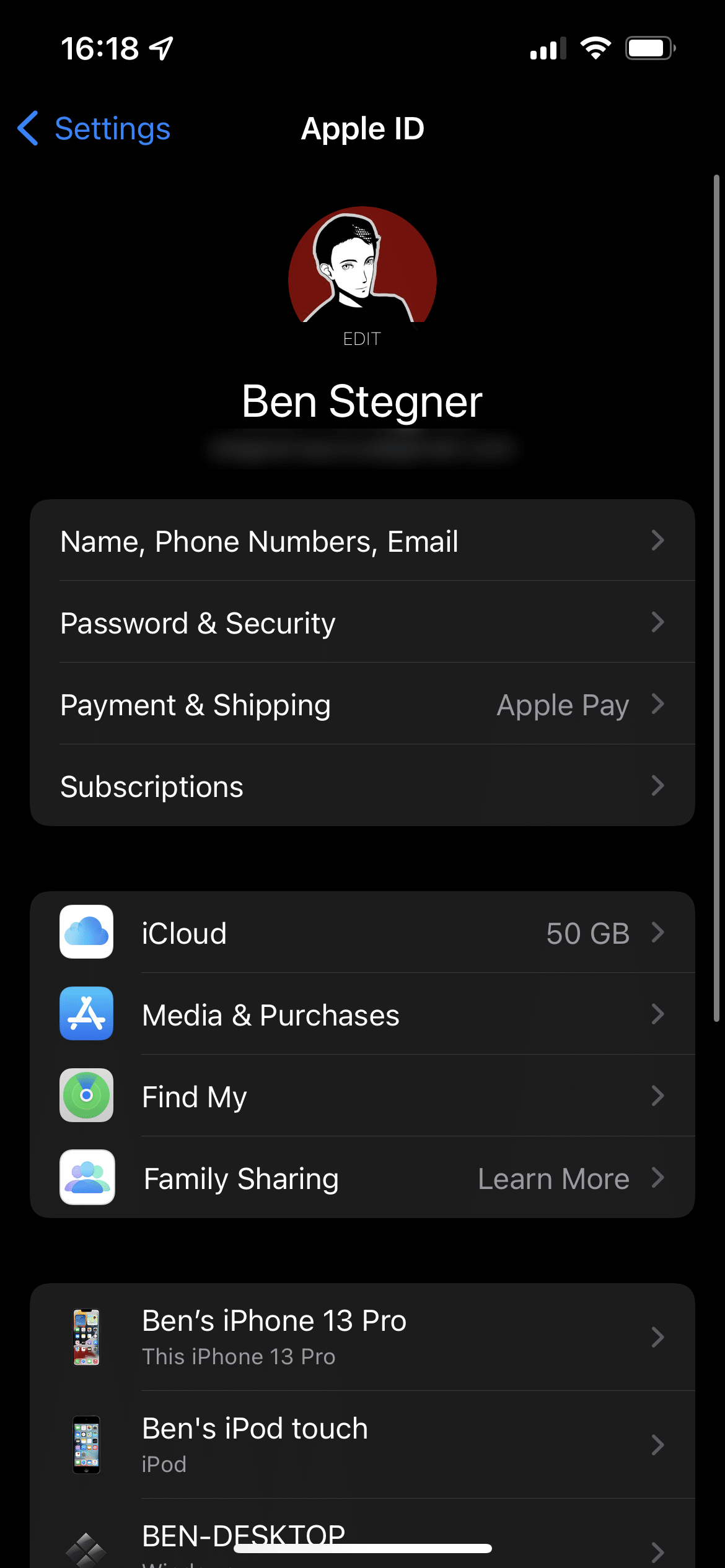The screenshot displays Ben Stegner's Apple ID information. His profile picture is a stylized black and white cartoon image set against a brown background. The screen is divided into four main sections: 

1. **Personal Information**: This section includes tabs for "Name, Phone Numbers, Email," followed by "Password and Security," "Payment and Shipping," and "Apple Pay" in grey text. Finally, "Subscriptions" is listed.

2. **Account Services**: Here, four app icons are shown: "iCloud," "Media and Purchases," "Find My," and "Family Sharing."

3. **Devices List**: A list of Ben's devices under his Apple ID includes "Ben's iPhone 13 Pro," "This iPhone 13 Pro (the device that captured the screenshot)," "Ben's iPod Touch," and "Ben's Desktop."

4. **Header Bar**: At the top-left corner, the current time is displayed as 16:18 (4:18 PM). The top-right corner shows three icons indicating network status (3 out of 4 bars), Wi-Fi signal strength (full at 3 out of 3 bars), and battery charge level (above 50%).

The summary offers a clear and detailed representation of Ben's Apple ID screen and associated information.